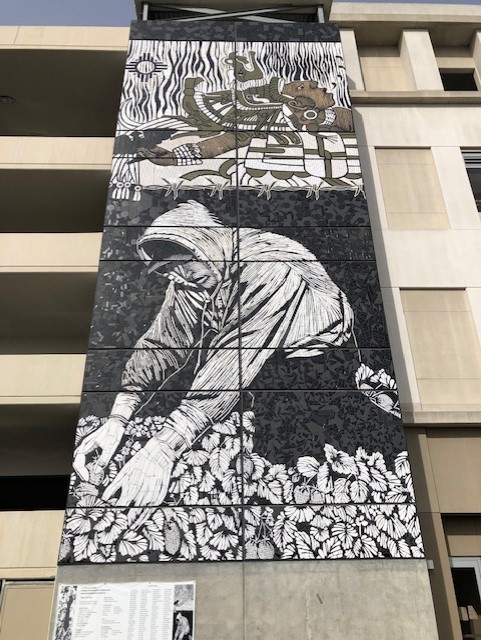The image showcases a detailed mural on the side of a neutral beige high-rise building, seemingly a parking garage, stretching across four to six stories. The mural is divided into two distinct sections with the top depiction featuring an indigenous figure, possibly Mesoamerican, illustrated in a blend of browns, blacks, and beige. The figure, whose skin is brown, wears a chieftain hat adorned with feathers and an interesting black and white garb. His head is tilted upward to the right, his eyes gazing skyward, and he holds a bird. There's a small sun sketch on the far upper level. Beneath this, the mural transitions predominantly to black and white, portraying a man in a hoodie and black baseball cap, engaged in gardening within a field of leaves. He's depicted on his knees wearing white gloves and dark pants, meticulously tending to the plants. The bottom two-thirds of the mural emphasize this monochromatic theme. A partially obscured informational plaque or poster is visible at the lower part of the building, potentially offering a description of the mural's imagery and significance.